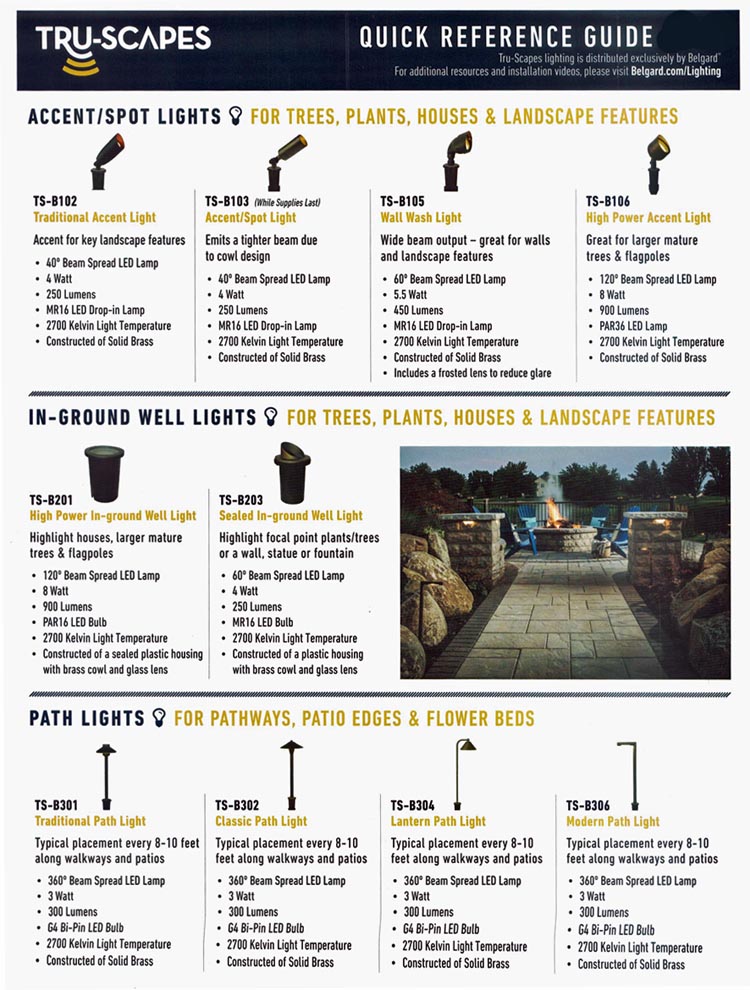This screenshot showcases the official TrueScapes website. At the top left corner, the header prominently displays the brand name "TrueScapes." The "True" portion of the logo is stylized as "T-R-U," where the "R" has an artistic curve extending beneath the "U," resembling a series of signal waves in vibrant orange. The title "Scapes" follows immediately after.

In the top right corner, the site provides a "Quick Reference Guide" in crisp white text. The central header of the page reads "TrueScapes Lighting," with a note underneath indicating that these products are exclusively distributed by Bellegarde. There's also an instructional note encouraging users to visit "bellegarde.com/lighting" for additional resources and installation videos.

The main body of the page promotes accent spotlights for various landscape features such as trees, plants, houses, and other elements. On the left, there is an image of a traditional accent light labeled "TS-B102," denoted as ideal for key landscape features, accompanied by a list of specific features for this particular light model. Adjacent to it, the other models "TS-B103," "TS-B105," and "TS-B106" are similarly displayed.

At the bottom right of the image, trash cans can be seen along with a variety of path lights, further illustrating the range of outdoor lighting solutions offered by TrueScapes.